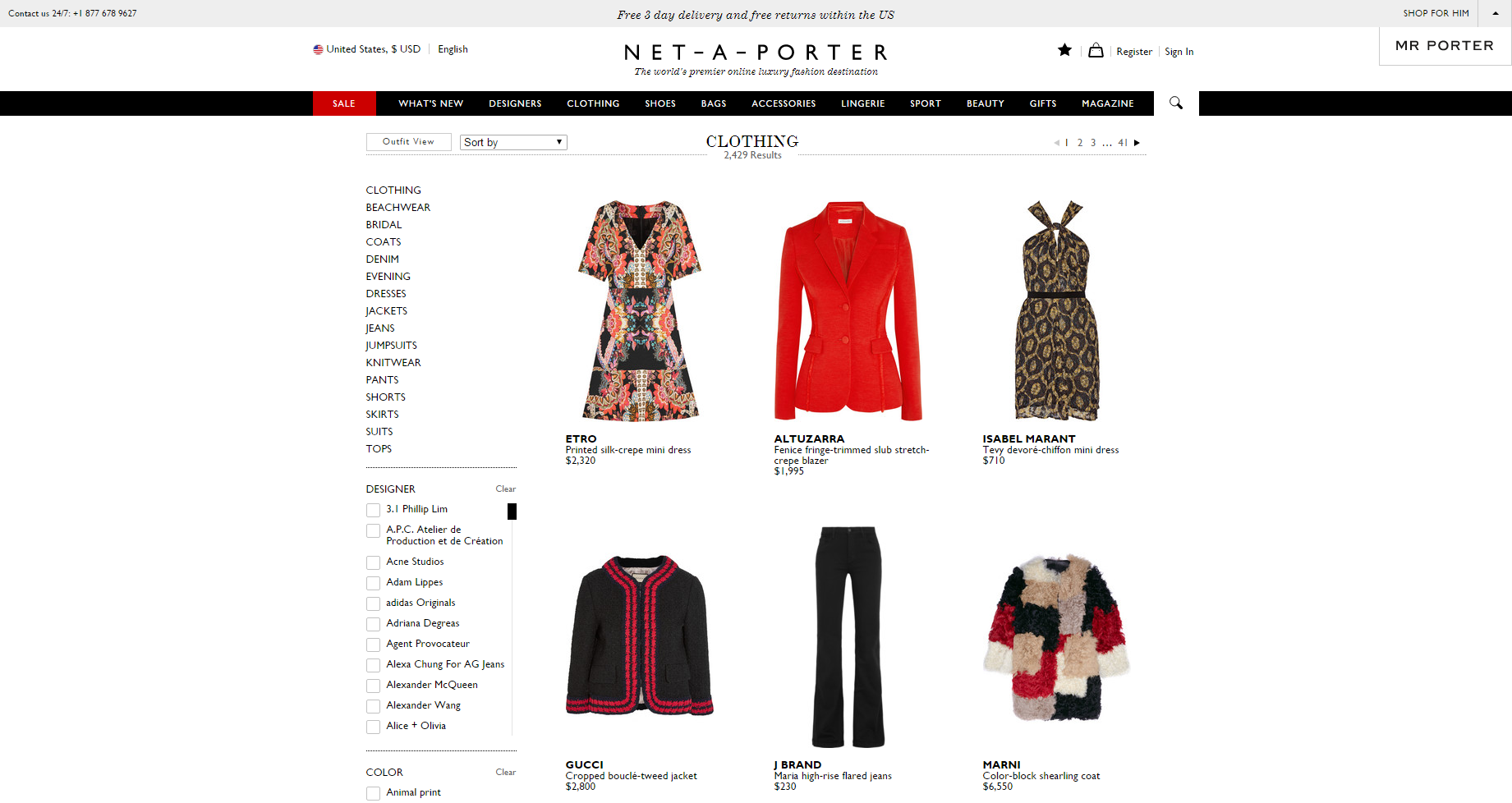The screen displays the homepage of Net-a-Porter, the world's premier online luxury fashion destination. At the top of the page, there is a prominent label stating "Free Three-Day Delivery and Free Returns Within the U.S." 

A sleek, black navigation bar runs across the width of the site, featuring menu options in white font: "Sale," "What's New," "Designers," "Clothing," "Shoes," "Bags," "Accessories," "Lingerie," "Sport," "Beauty," "Gifts," and "Magazine." The "Sale" option stands out with a red background and white font. To the right of the menu options is a search icon represented by a magnifying glass.

Below the navigation bar, there is a list of category options on the left side, including "Clothing," "Beachwear," "Bridal," "Coats," "Denim," "Evening Dresses," "Jackets," "Jeans," "Jumpsuits," "Knitwear," "Pants," "Shorts," "Shirts," "Skirts," "Suits," "Tops," and more, followed by a line and a list of different designers to choose from.

In the main content area, there is a "Sort By" drop-down menu, an indication of "Clothing – 2429 results," and pagination links starting with "1, 2, 3 ... 41." The products are displayed in a grid format, with three items per row, and two rows visible on the screen.